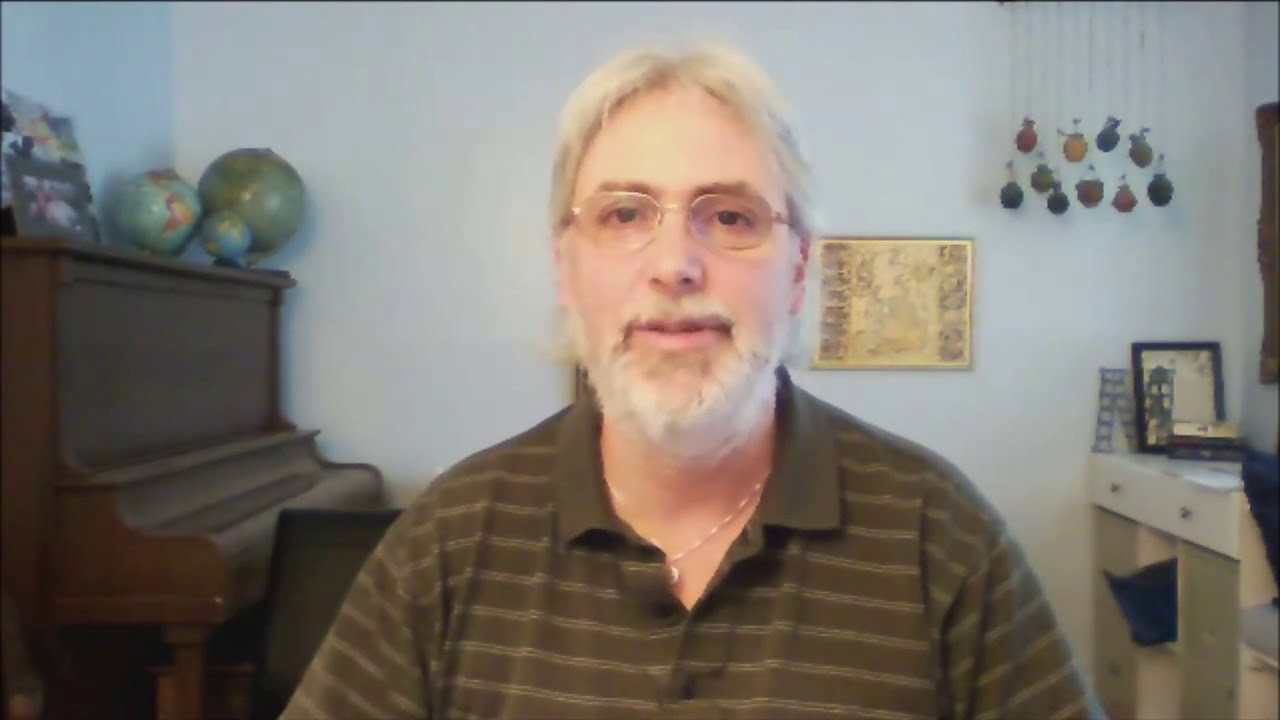The image depicts an older white man with white hair, a white beard, and a white mustache, wearing clear glasses. He is seated and facing the camera, possibly during a web meeting. He is dressed in an olive green, collared shirt with white stripes and a gold necklace. His expression suggests he may be engaging in conversation. 

The background of the room features a light blue wall intersecting with a slightly darker blue wall. Against the left wall stands a brown piano topped with three globes and a book or portrait leaning against the wall. To the right of the man is a shelving unit or dresser with two drawers at the top and shelves below, holding various picture frames and books. Additionally, there is a map on the wall and a tapestry with egg-shaped objects hanging on the top right. A mobile with round objects in blue, red, yellow, and green hues hangs from the ceiling. The detailed setup of the room, along with the man's appearance, creates an inviting and intellectual atmosphere.